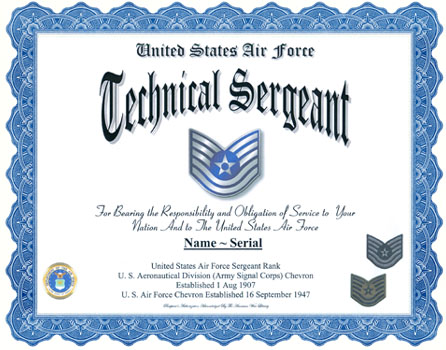This image depicts a certificate from the United States Air Force, distinguished by an intricate blue border adorned with circular patterns. At the top center, stylized calligraphy reads "United States Air Force," followed by "Technical Sergeant" in prominent, larger letters. Below this is a crest featuring a star at its center.

The certificate’s text elaborates further, in cursive: "For bearing the responsibility and obligation of service to your nation and to the United States Air Force." Lower still, in standard font, placeholders marked "Name" and "Serial" are underlined, indicating where personalized details would be entered. The certificate continues with historical context: "United States Air Force Sergeant Rank," followed by "U.S. Aeronautical Division [Army Signal Corps]," and importantly, notes the establishment dates, "Chevron established 1 AUG 1907" and "U.S. Air Force Chevron established 16 September 1947."

At the bottom left is the United States seal, and the bottom right features a logo similar to the crest in the center, likely representing the United States Air Force. The certificate is clearly a template awaiting personalization for its intended recipient.